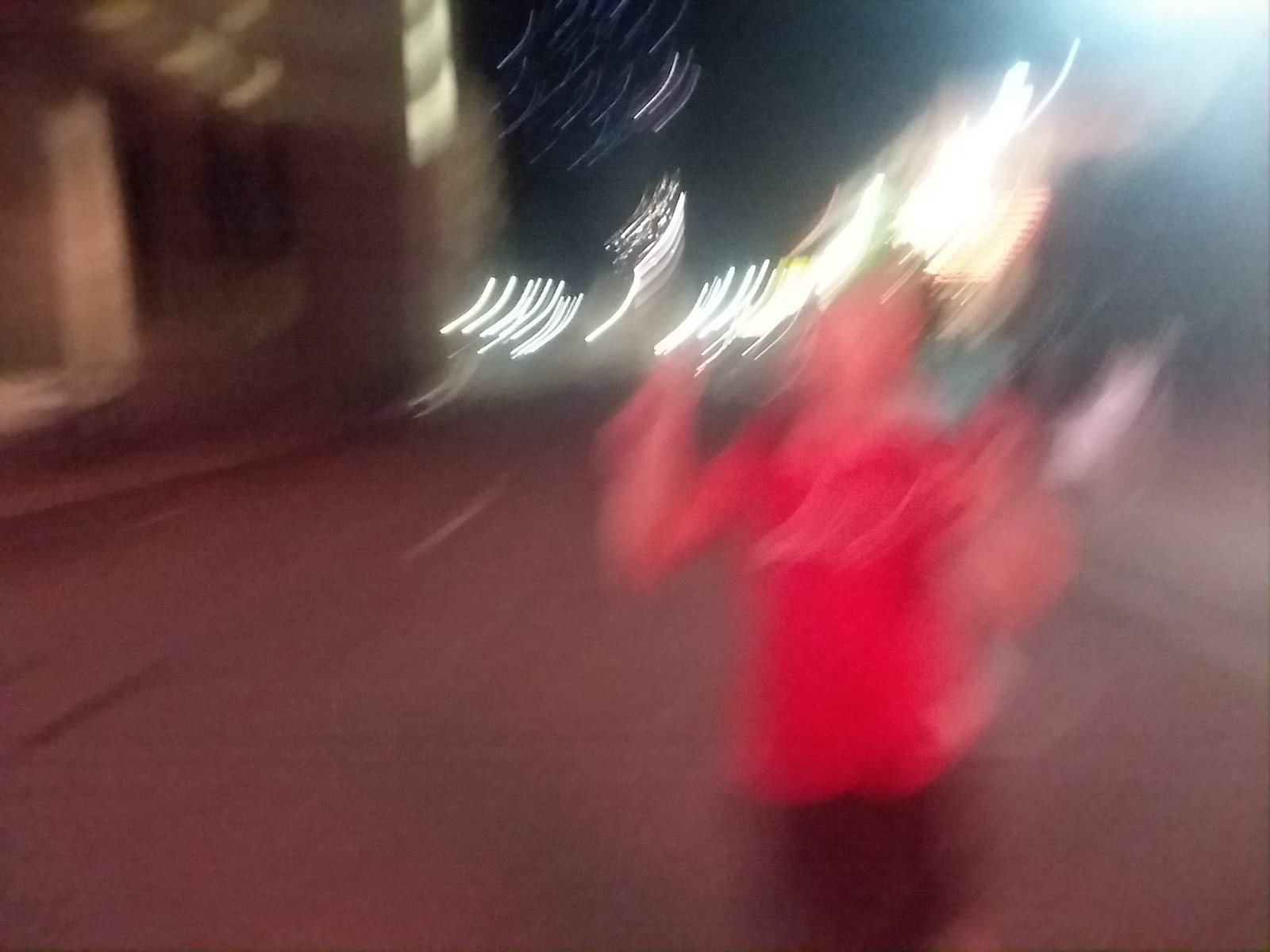A blurry nighttime photograph captures the dynamic motion of an individual wearing a red shirt and brown pants, seemingly presenting an object with both hands towards the camera. However, the motion blur obscures the details of the object. The background reveals a road with white lines in the middle, hinting at a black asphalt surface. A building stands to the left, faintly illuminated by several lights. The lights, like streaks, show a consistent jerking motion, indicating that the camera was shaken at the moment the photo was taken, adding to the overall sense of movement and obscurity in the image.